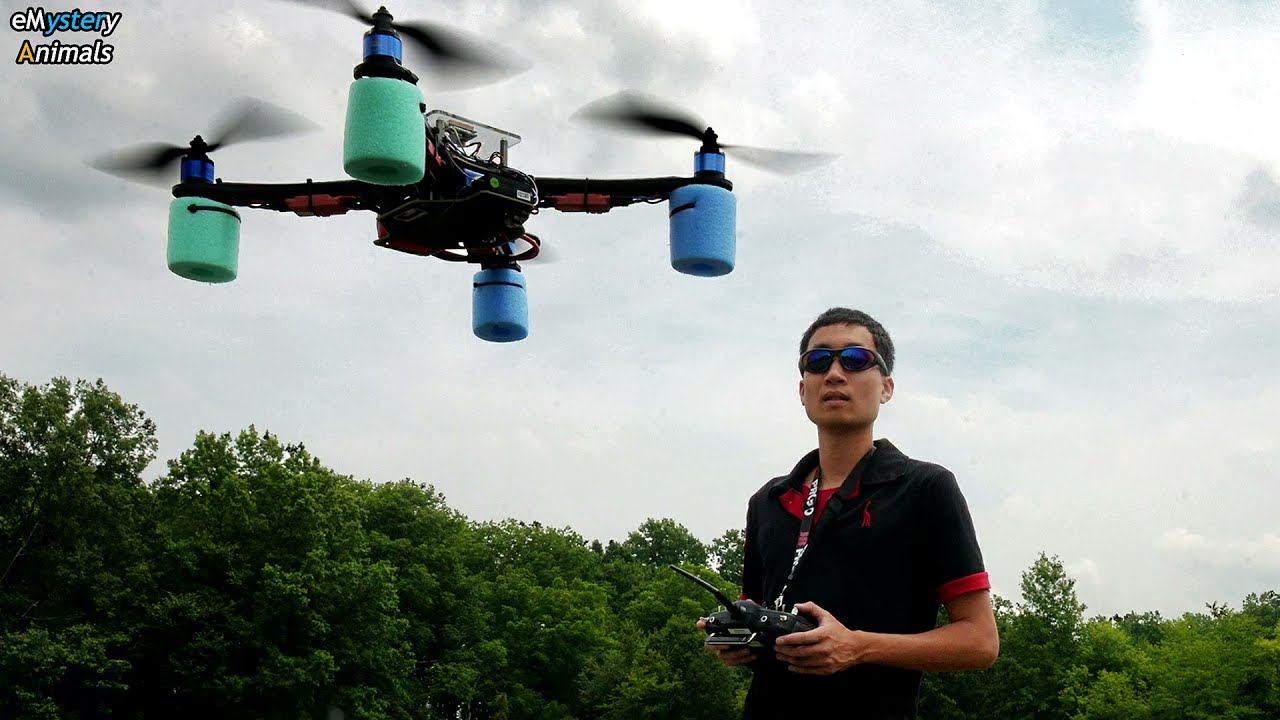In this photograph, a young man is seen operating a large drone using a remote control. The man, who is of Asian descent, is standing outdoors in front of a row of green shrubs or trees. The sky above is cloudy, yet it appears to be a sunny day. The drone, which is captured in the upper left corner of the image, is wrapped with green and blue foam around the points of its propellers. This foam might serve to protect the drone during landings or improve its aerodynamics. The man is dressed in a black polo shirt with a visible red undershirt and a red logo on his chest. He is also wearing mirrored dark sunglasses, adding a touch of modernity to his appearance. He holds the drone’s remote control firmly with both hands as he navigates the device through the air, offering a glimpse into a recreational or perhaps experimental remote control flying session.